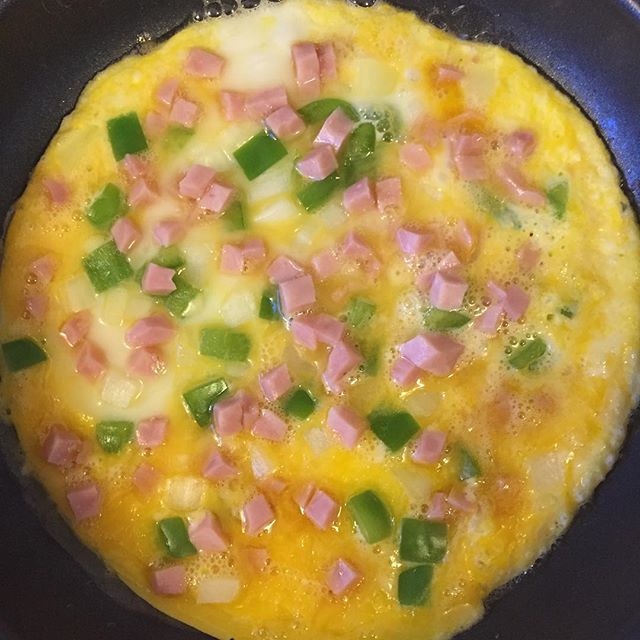This vivid, square photograph captures a top-down, close-up view of an omelette cooking in a black skillet. The omelette, still not fully set, appears slightly runny with bubbling edges, where the oil in the pan shimmers. The egg mixture comprises about three eggs, a blend of yellow yolks and whites, mingling together. Small, evenly distributed pieces of diced ham, green bell pepper, and possibly some light onions are visibly scattered across the omelette. The ingredients create a well-balanced mosaic atop the nearly solidified egg layer, suggesting the omelette is nearly ready to flip. The surrounding black edge of the skillet frames the circular dish, emphasizing its appetizing colors and texture in the cooking process.